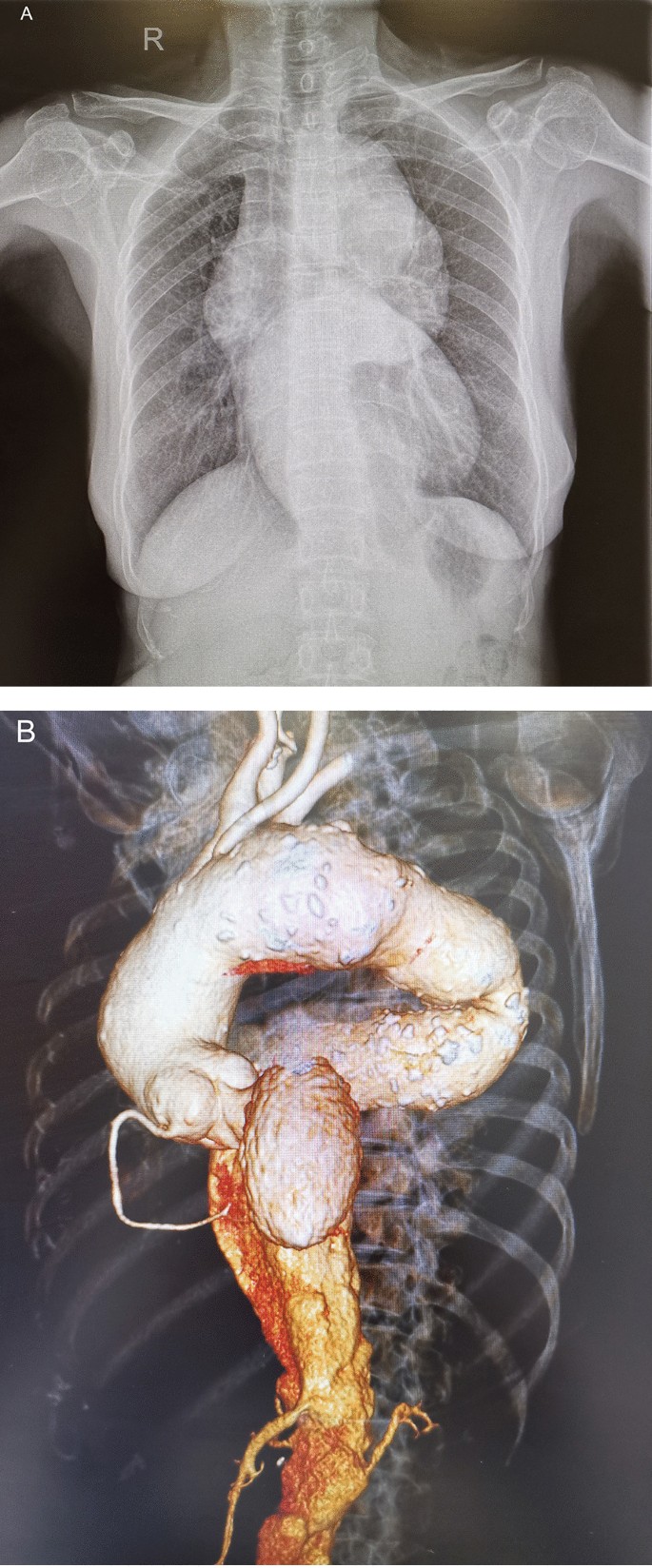The provided image comprises two distinct medical scans, labeled A and B, displayed one above the other in a column. The top image, designated as A, is a black-and-white x-ray of a human torso, extending from the neck to the stomach. This x-ray reveals the skeletal structure, including the clavicles, ribcage, shoulder blades, and spine, which are all clearly visible. The organs within the chest and abdomen, although faint, can also be observed, offering a standard radiographic view.

The bottom image, labeled B, is a more advanced 3D imaging scan that conveys a detailed and colored representation of the same region. In this scan, the skeletal outline remains visible but serves as a backdrop to the prominently featured internal organs. These organs are vividly colored, transitioning from white at the top to shades of red, yellow, and orange, highlighting various anatomical structures and potentially pathological areas. The scan suggests a significant deformation, possibly indicative of a tumorous or cancerous growth, particularly a striking orange-to-yellow mass extending from the upper section to the bottom center. This detailed imagery in B provides a more comprehensive anatomical perspective than the x-ray in A, aiding in the diagnosis.